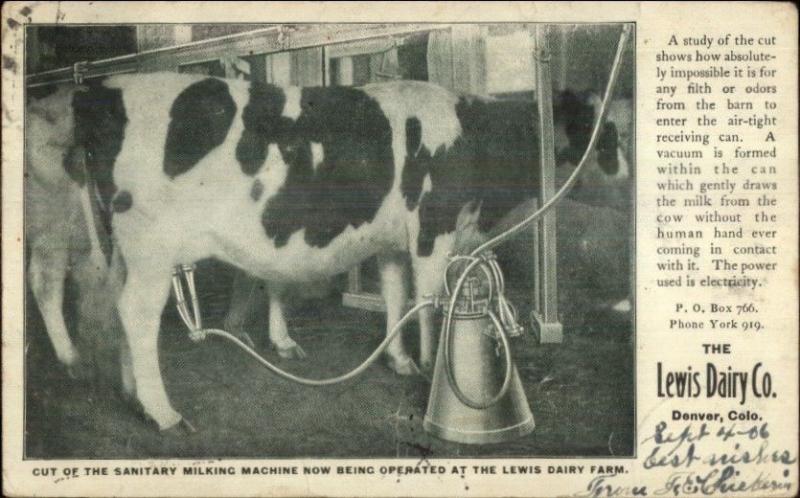The image depicts an old newspaper clipping featuring a black and white photograph of a barn interior with a dairy cow hooked up to a shiny, sanitary milking machine. The machine has tubes connected to the cow’s teats and extending to the upper right part of the image. Below the photograph, a caption reads: "Cut of the sanitary milking machine now being operated at the Lewis Dairy Farm." The article text on the right elaborates on the machinery, stating, "A study of the cut shows how absolutely impossible it is for any filth or odors from the barn to enter the airtight receiving can. A vacuum is formed within the can which gently draws the milk from the cow without the human hand ever coming in contact with it. The power used is electricity." Additional information includes, "P.O. Box 766, Phone York 919," and it’s from "The Lewis Dairy Company, Denver, Colorado." There is also some handwritten text in the bottom right corner, though it is not completely legible, mentioning "September" and "best wishes." The background of the clipping has smudges indicative of its age.